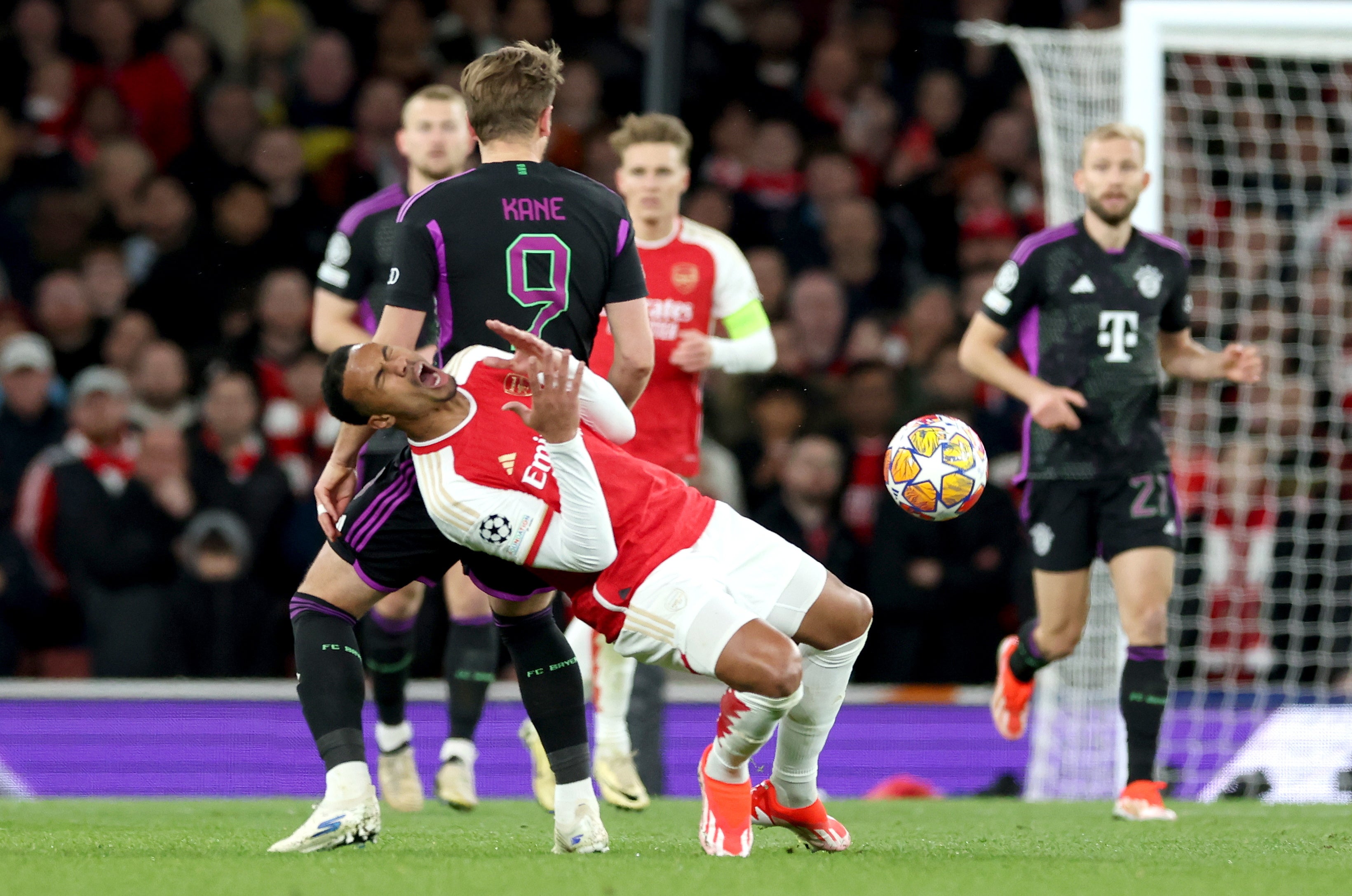In the foreground of the image, a dynamic scene of a soccer match unfolds on a lush, green field. The central focus is on a player clad in red and white who appears to be in the process of falling, his body mid-motion, an embodiment of the sport's intense physicality. Nearby, a soccer ball is suspended in midair, capturing the quintessential moment of action. Surrounding him are teammates and opponents: one player in identical red and white uniform, while two adversaries don black and purple attire, adding a stark contrast. Off to the right, a large white net stands prominently, with another player in black and purple stationed near it, likely the goalkeeper. In the background, a blurry crowd watches intently, their indistinct figures adding a backdrop of excitement and anticipation to the scene.